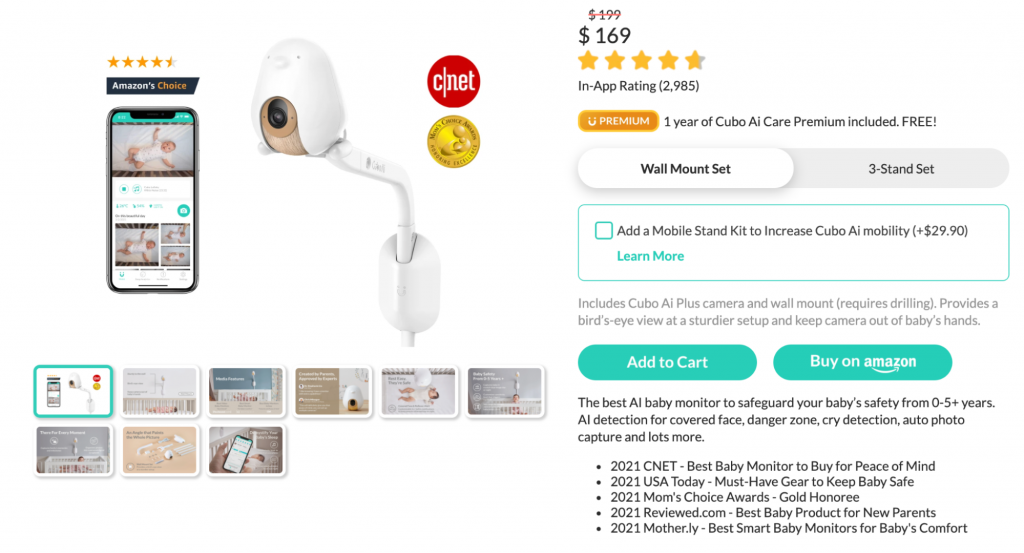The screenshot showcases a product listing on the CNET website for a versatile baby monitor camera, designed for parental convenience and security. On the left side of the screen, the product features an impressive 4.5-star rating, prominently displayed alongside an "Amazon's Choice" badge, which consists of a white "Amazon" text paired with a gold "Choice" label. Beneath these accolades, an icon of a smartphone highlights that the webcam's feed can be accessed through a mobile app.

The main image carousel offers various views of the camera, including top-down and side angles, illustrating its robust functionality. The camera itself is shown mounted on a flexible arm capable of pivoting and twisting in multiple directions, ensuring comprehensive coverage of your baby's environment. Adjacent to the smartphone icon, a gold seal announces the camera as "Baby and Pediatrician Approved," while a red circular tag indicates the CNET endorsement.

Below the primary camera depiction, several icons provide quick access to more detailed information about the webcam's features, such as interactive video options for voice and recording capabilities. The right section of the page supplies essential purchasing details, highlighting a discounted price: originally $199, now $169. Alongside this, there are in-app reviews totaling 2,985, averaging to a 4.5-star rating.

Potential buyers are presented with multiple purchasing options, including a wall mount set (default checked) and a three-stand set (unchecked). An optional mobile stand kit, enhancing Qubo AI's portability, is available for an additional $2,990. The listing further promotes a premium service, indicating that one year of Qubo AI care premium is included for free.

Additionally, shoppers can add the item to their cart or choose to buy it directly on Amazon. The page concludes with a description of various awards the baby monitor has garnered, solidifying its reputation as a reliable and award-winning product.